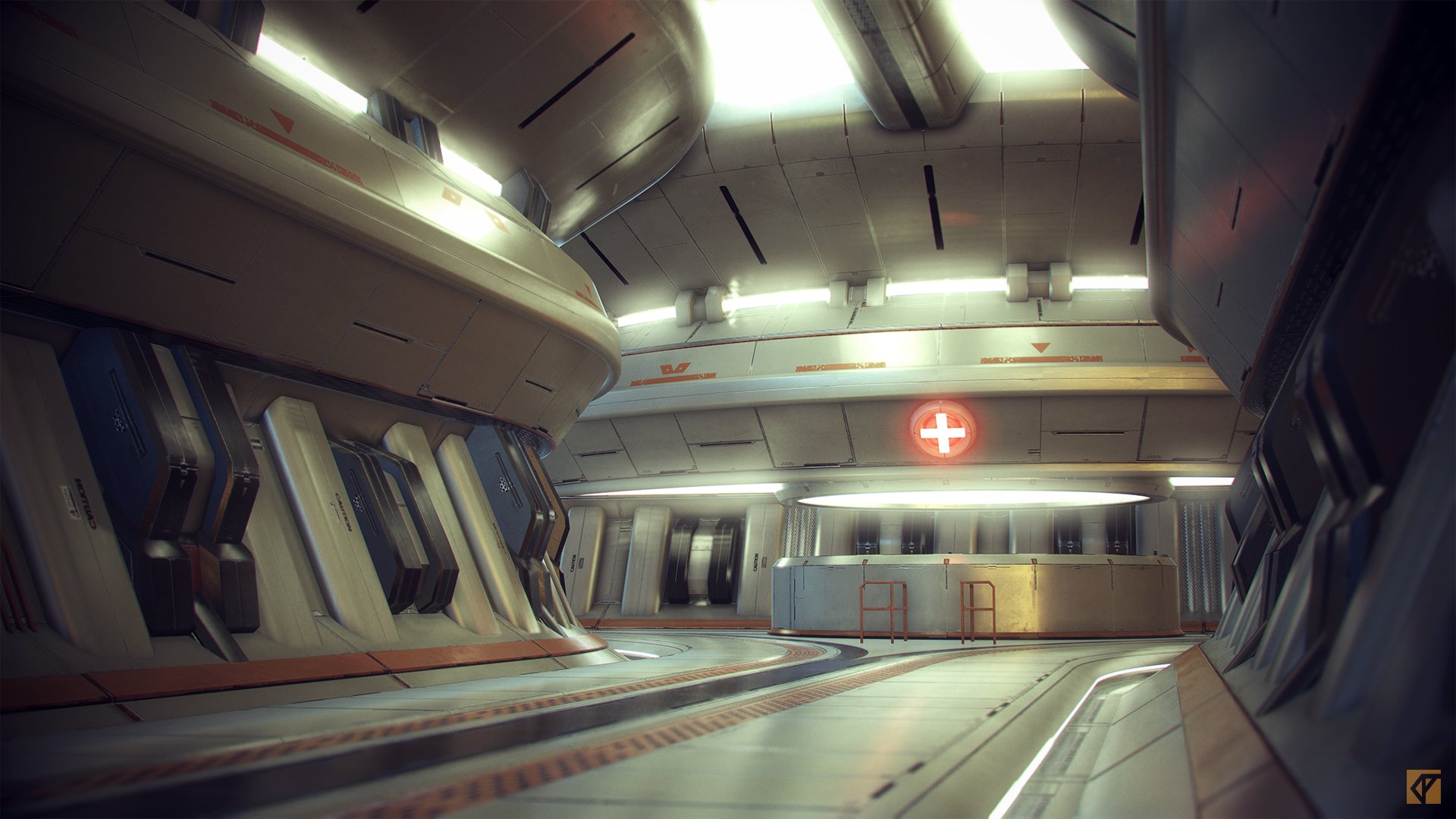The image depicts the interior of a futuristic, possibly subterranean, transport system or spaceship. A wide corridor features tracks running along one side, flanked by curved white and black walls adorned with various built-in elements. The walls and overall structure curve to both the left and right beyond a prominent round desk. This desk is illuminated by a large white light above it, and a striking red circle with a white cross hangs over it, suggesting an emergency or medical station. The corridor is also equipped with skylights above, flooding the space with daylight. Black, curved windows line the walls, adding to the high-tech aesthetic. There are also red railings in front of the desk, which further emphasizes the organized nature of the space. Complex markings are scattered throughout the structure, hinting at its advanced functionality.